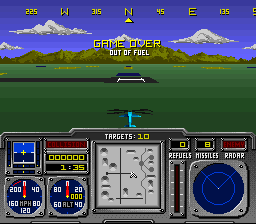This image is a square digital snapshot from an older video game, likely from the 1980s or early 1990s given its low-detail graphics. At the bottom of the screen, there is a detailed control panel, suggesting the perspective is from inside a cockpit. This panel includes numerous dials, a radar display, and a small propeller protruding from the front of a gray dashboard. The green field extending beyond the cockpit might represent the ground or surrounding terrain. On the left side, a landing pad is just coming into view, shrouded in darkness. The backdrop features a mountain range overlaid with the text "GAME OVER, OUT OF FUEL." A top banner displays "WNE," potentially indicating navigational directions. The color scheme is a mix of blues, yellows, reds, greens, whites, and browns, contributing to the nostalgic aesthetic of the game.